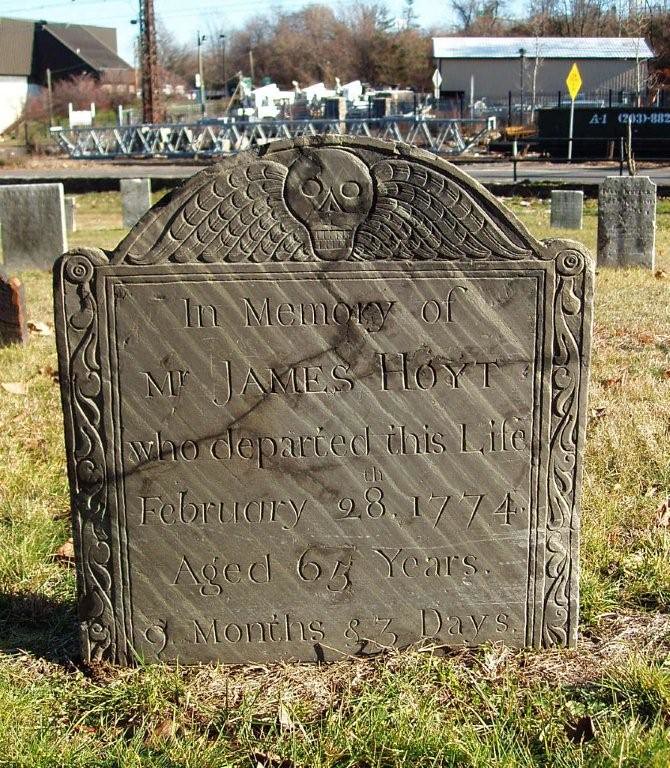This full-color photograph captures a gravestone in an outdoor cemetery, taken likely during fall or spring as suggested by the leafless trees and the clear daytime sky. The headstone, a brownish stone, is intricately carved with ornate details, featuring a human skull with wings on top. It memorializes Mr. James Hoyt, who departed this life on February 28, 1774, aged 65 years, 9 months, and 3 days. The gravestone, exceptionally well-preserved for nearly 250 years, stands in contrast to its surroundings. Behind the cemetery, across the street, lies an industrial area with various machines and outbuildings. On the left, a brown building and tower can be seen, while to the right, a silvery metallic structure is noticeable along with a yellow street sign. The scene also includes what appears to be a stage or some setup in the background, adding a layer of modern juxtaposition to the historical site.